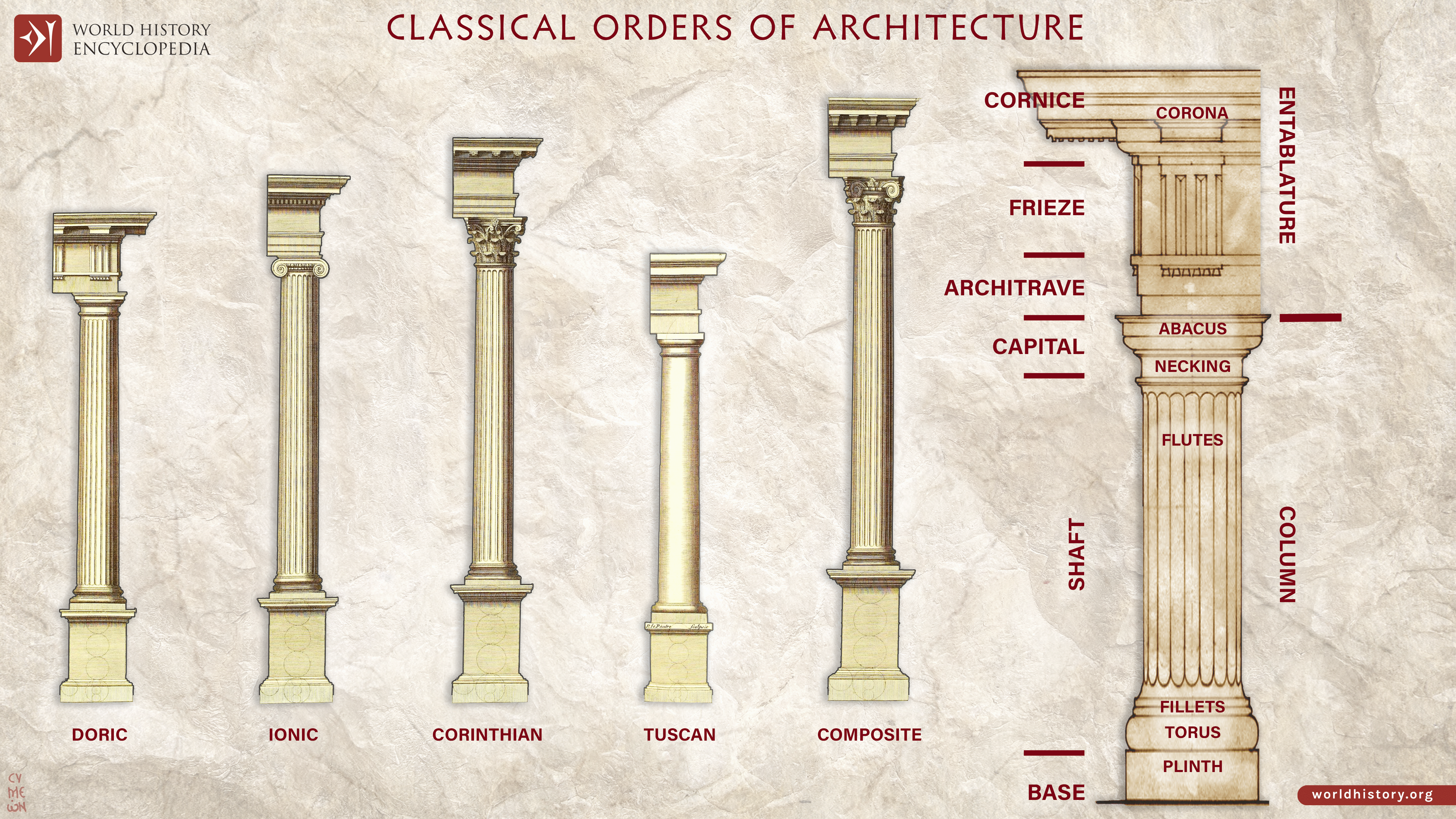This image is a detailed diagram from the World History Encyclopedia, showing the evolution of the classical orders of architecture. The background features a stone-like pattern, enhancing its historical appearance. At the top left corner, there is a red square logo with white symbols, accompanied by the text "World History Encyclopedia." The bottom right corner contains a similar red box that reads "worldhistory.org."

Prominently displayed at the top center of the image, in a Greek-style font, are the words "Classical Orders of Architecture." Below this header, six cream-colored architectural columns stand in sequence against a white, crumpled-paper background, each representing a different classical order: Doric, Ionic, Corinthian, Tuscan, Composite, and a labeled diagram of the column's parts. The Doric order, known for its simplicity, is distinguished by its sturdy form and plain capital. The Ionic order is taller with a narrow top. The Corinthian order features more elaborate decorations at both the top and bottom. The Tuscan order is similar but smoother and smaller. The Composite order is the tallest and often the most ornate. 

To the far right of these columns, there is a detailed breakdown of a column’s components, including the base, plinth, torus, shaft, fillet, necking, cornice, and corona. This comprehensive illustration provides an informative guide to the classical architectural styles that have shaped historical and modern designs.